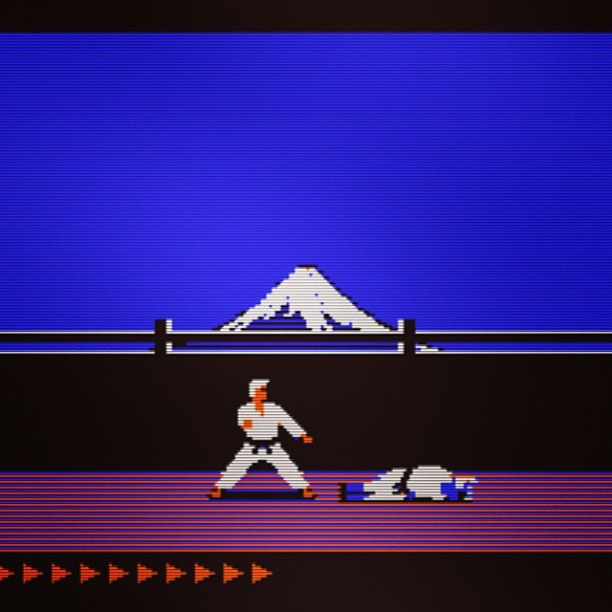This screenshot of an early 90s or 2000s Nintendo SNES-era video game captures a classic fight scene within a rudimentary graphic environment characteristic of old-style video games. The image prominently features two characters on what appears to be a balcony setting with a blue sky and snow-capped conical mountaintop in the background, framed by a black wall and railing. The foreground showcases a fighting platform with alternating orange and blue horizontal stripes. 

The main action unfolds in the lower third of the frame, where one character is seen in a karate stance facing right. This character is in a white long-sleeved top and trousers, displaying a black belt with its ends pointing diagonally downwards, and has orangish skin tone for his hands and feet. Another character, similarly clad in white attire with a black belt, lies on the floor to the right, featuring blue skin tone. Additionally, the screen’s bottom black border is populated by ten red arrows pointing to the right, possibly indicating game instructions or direction, although it is partially cut off on the left side. The screen's visual style, complete with horizontal lines reminiscent of a cathode ray tube television, enhances the nostalgic old-school gaming experience.